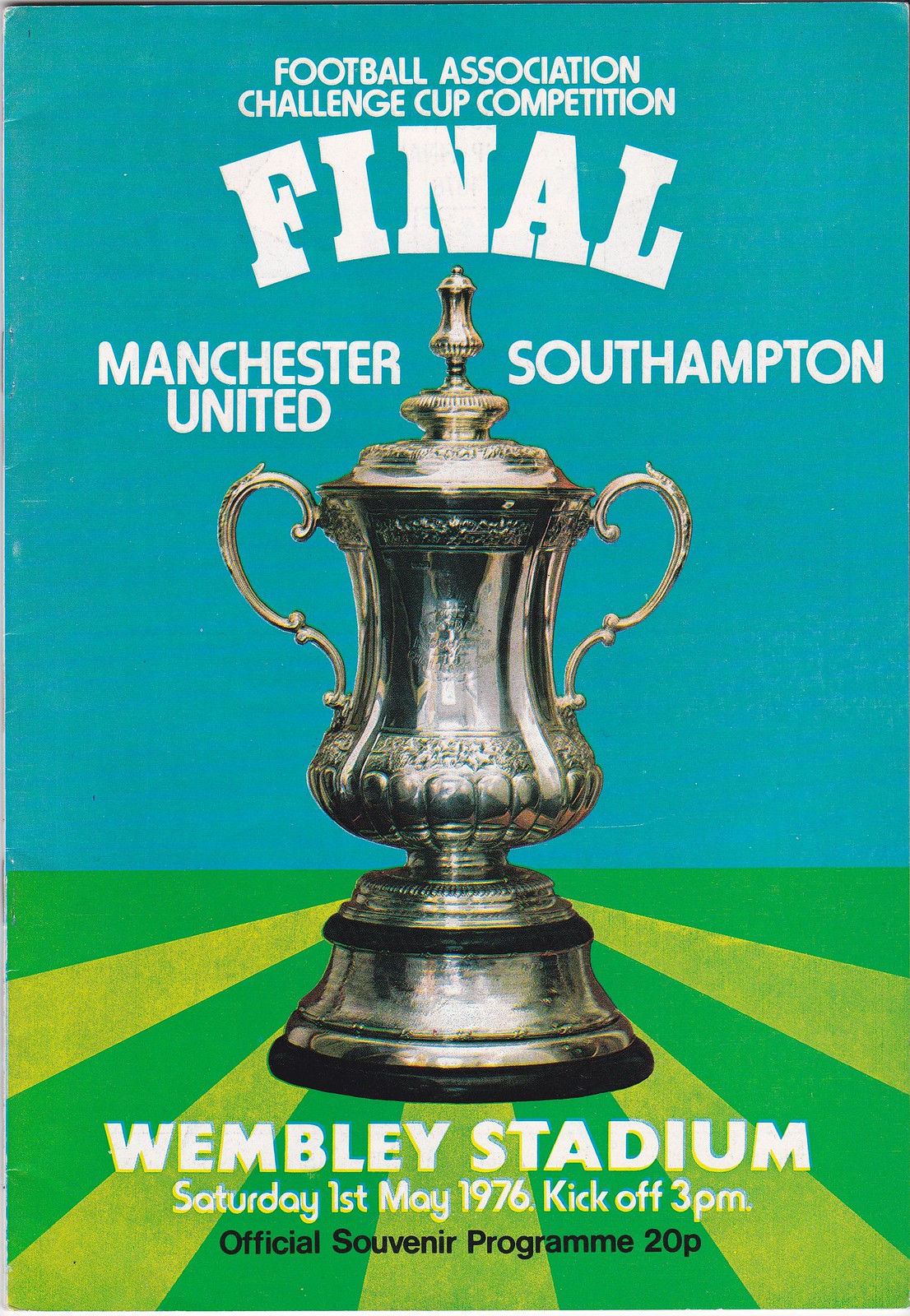This detailed poster, advertising a soccer championship match, features a prominent silver trophy placed centrally. The top section of the image has a solid teal background and contains the title in bold white letters: "Football Association Challenge Cup Competition Final." Flanking the trophy are the team names "Manchester United" and "Southampton." The bottom third of the poster transitions into a background with green and yellow sunburst stripes emanating from the center. Below the trophy, white text announces the venue and details: "Wembley Stadium, Saturday 1st May 1976, kick-off 3 p.m." The final detail, in smaller black text, reads "Official Souvenir Programme 20P."